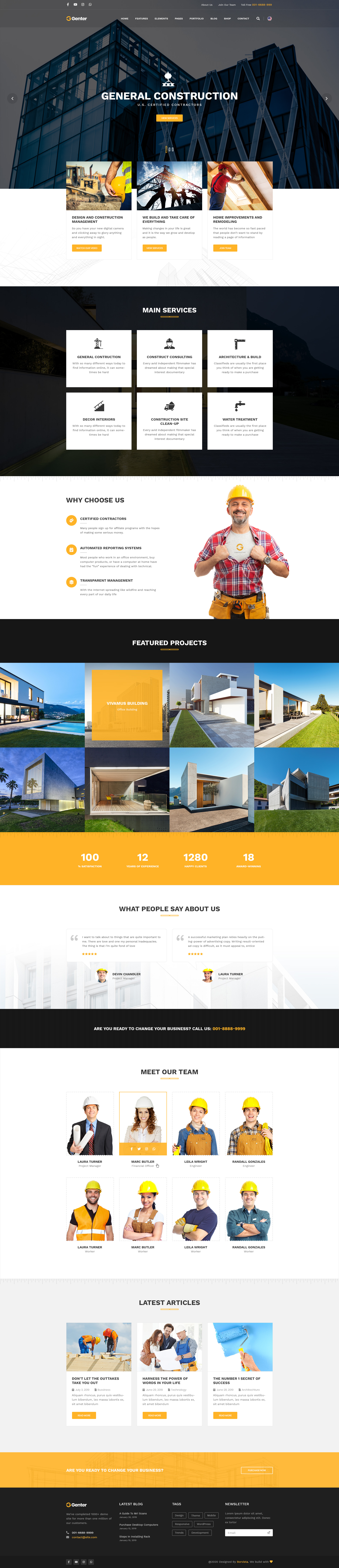The image appears to be an elongated, stitched-together version of a construction company's webpage, capturing various sections from top to bottom.

At the top of the page, there are categories and tabs related to general construction, though the exact names and the company’s logo are not readable. This section includes three pictures: one of a gentleman at a construction yard, several construction workers, and another person working with wood. The backdrop features a large, modern glass and metal structure.

The next section, which seems to outline the company's services, includes an image of a man in construction attire—plaid shirt, worker's belt, and yellow hard hat. The text includes a segment titled "Why Choose Us," although the specific reasons are unclear.

Midway down the page, there's a section showcasing "Featured Projects." This part displays images of contemporary homes, possibly located in beachfront settings. The text mentions something about completing 100+ projects and includes a "What People Say About Us" segment with two testimonials, though the specifics are illegible.

Further down, there’s a "Meet Our Team" section featuring eight individuals in hard hats. Highlighted is a woman in a white hard hat and a pantsuit. To the left stands a man in a suit and tie, and next to him are a man and woman in overalls and yellow hard hats. The remaining four individuals include a man with a beard in a yellow safety vest, a woman in brown overalls and a yellow hard hat, a man in a blue shirt, and another in an aqua-green shirt.

The final segment highlights the "Latest Articles," likely news related to the construction industry, followed by the standard "Contact Us" information with email and contact details at the very bottom.